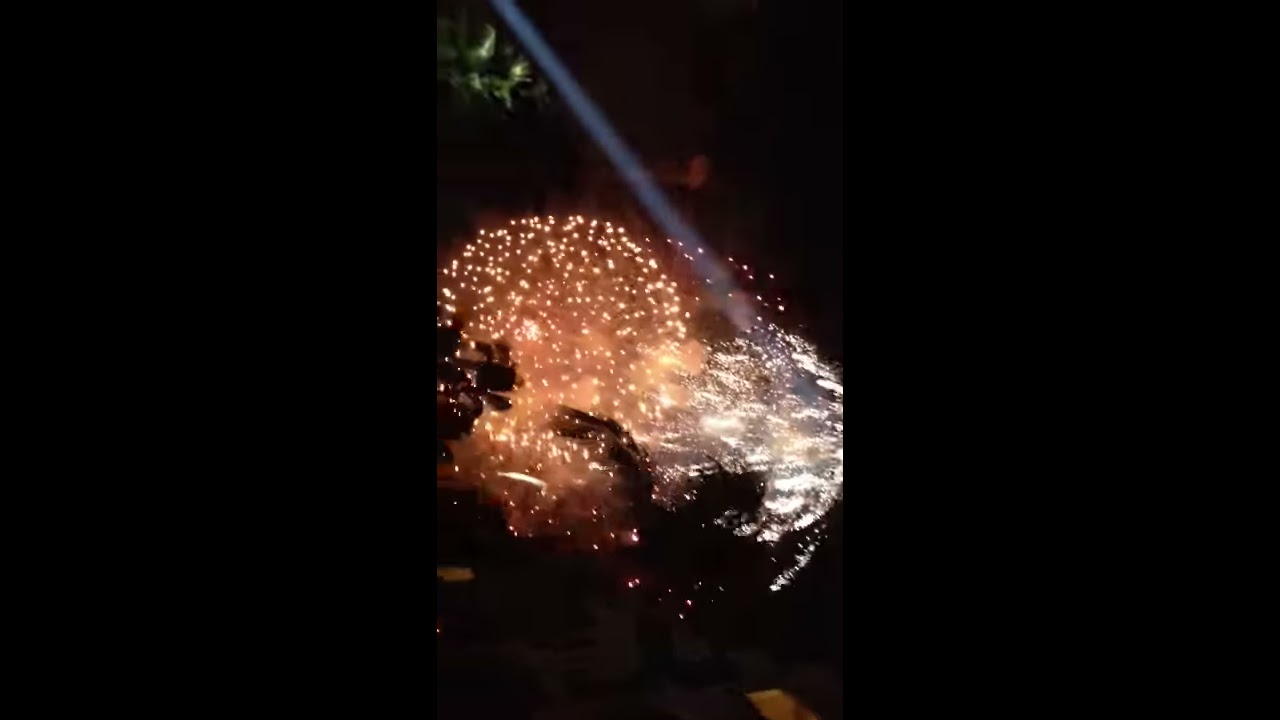The image is divided into three vertical sections, with the left and right thirds being solid black. Dominating the center section are bright lights which appear to be two fireworks exploding in the sky. The background remains a plain black, providing contrast to the vivid lights. 

On the right side, at the halfway point, a spherical burst of elongated, horizontal white lights radiates, suggesting a firework launched from that side. The central area features a spherical cluster of small, orangish-red lights, accompanied by an orange-tinted dust cloud. These lights are complemented by shadows and branches of trees silhouetted against the glow. From the upper left corner, a small beam of bluish light shoots down diagonally toward the right, where more greenish lights are visible, adding varied color to the scene. The detailed interplay of lights and shadows creates a dynamic and captivating visual experience, illuminated further by a dense scatter of orange dots on the left side and an intense white-blue explosion on the right.